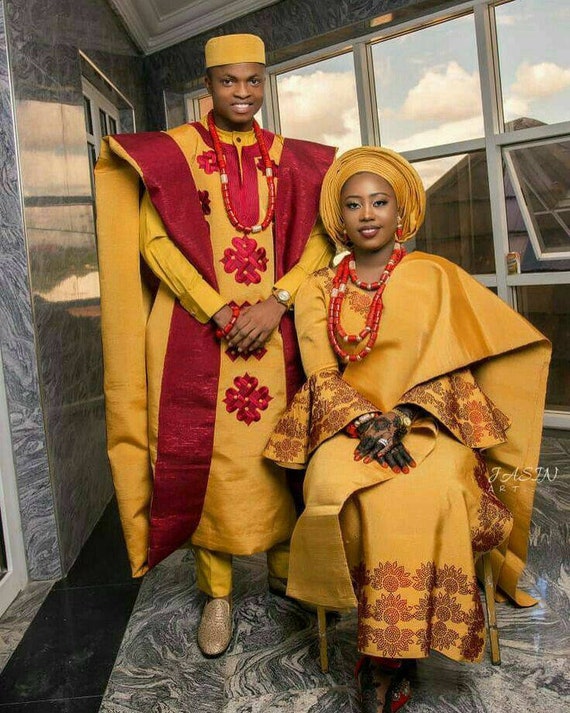The photograph depicts an African couple adorned in traditional wedding attire, predominantly yellow with intricate red detailing. The man, standing to the left, wears a cap and a garb with red clover patterns along with gray shoes. His vibrant outfit includes a massive red necklace and red detailing, akin to a comforter draped straight down. He also accessorizes with a red bracelet on his right wrist, and a watch on his left. The woman seated beside him, dressed in a matching gold-colored ensemble, wears multiple long red necklaces and a headdress resembling a sun hat. Both are smiling warmly at the camera, their teeth visible. They are situated in a large room with numerous square windows behind them, one of which is open. The room features dark marble with black swirls and granite flooring, adding to its grand ambiance.